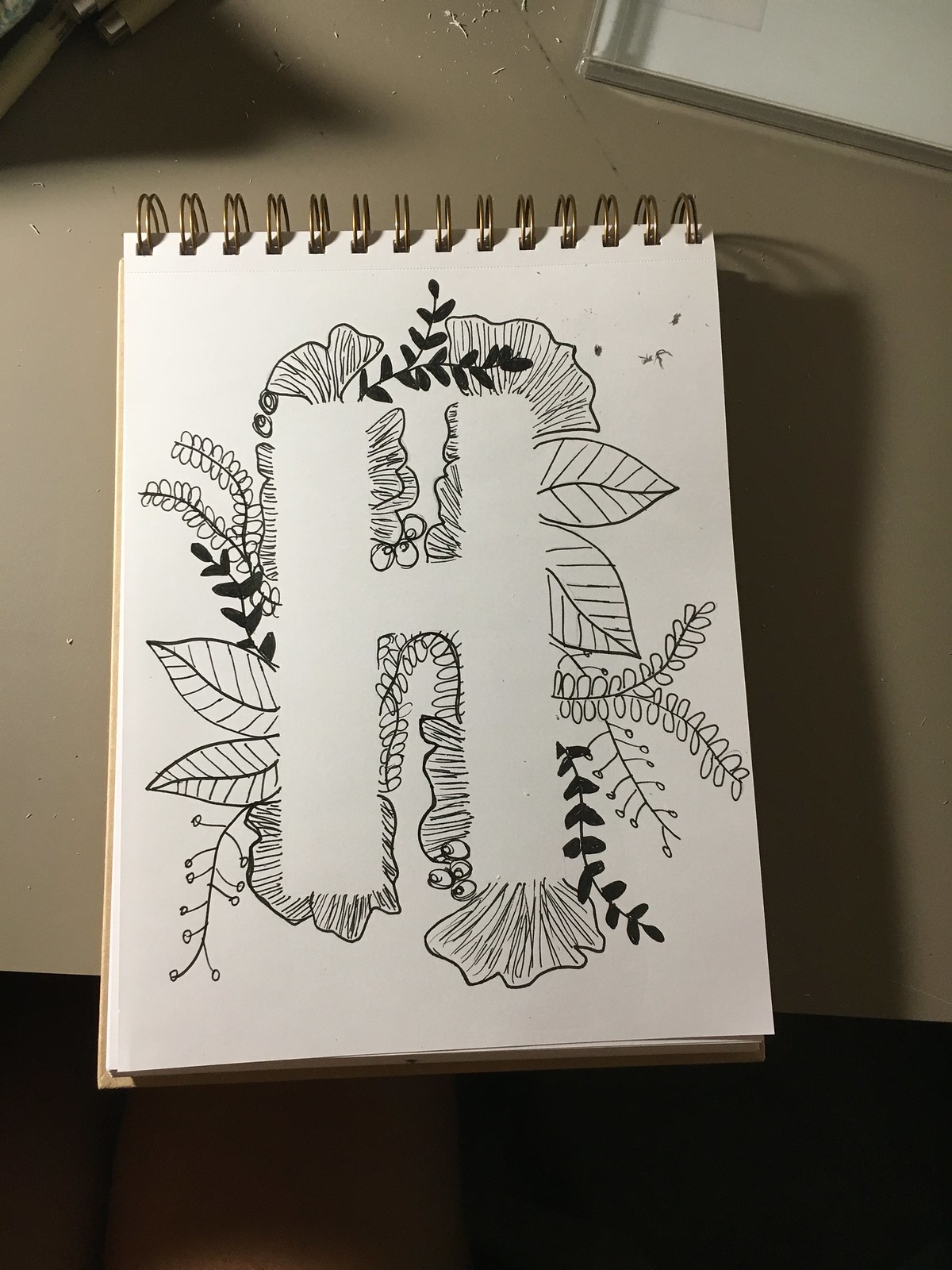This indoor photograph captures a close-up view of a spiral-bound art notepad resting on a gray desk. The notepad's spiral binding can be seen clearly at the top of the page. The artist has intricately drawn a floral design across the entire page, skillfully leaving the prominent shape of a capital "H" blank in the center. The "H" stands out against the detailed background of flowers surrounding it, creating a striking and creative contrast.